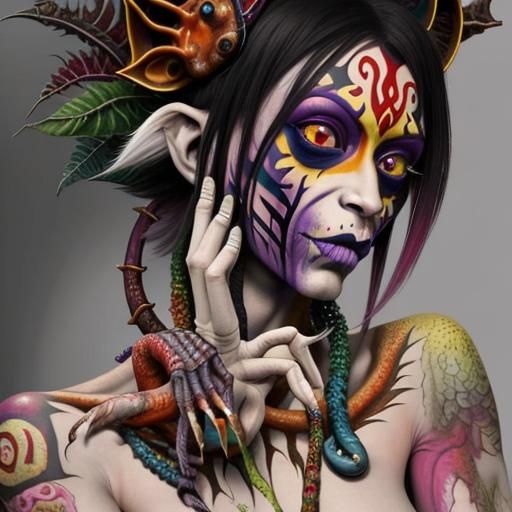This image showcases a highly realistic, computer-generated avatar resembling a female figure. The avatar features striking, yellow eyes with red pupils, creating an intense gaze. Her face is adorned with a blend of intricate tattoos and elaborate face paints, adding an otherworldly charm to her appearance. Jet-black hair frames her face, interspersed with floral and plant-like designs, and a distinctive streak of white hair flows back over her right ear. Around her neck, an optical illusion of intertwined vines and hands gives the impression of wings and adds to the surreal, ethereal quality of her design. Her arms are elaborately tattooed with vibrant colors, including shades of pink, yellow, and red, enhancing the avatar's detailed and captivating aesthetic.